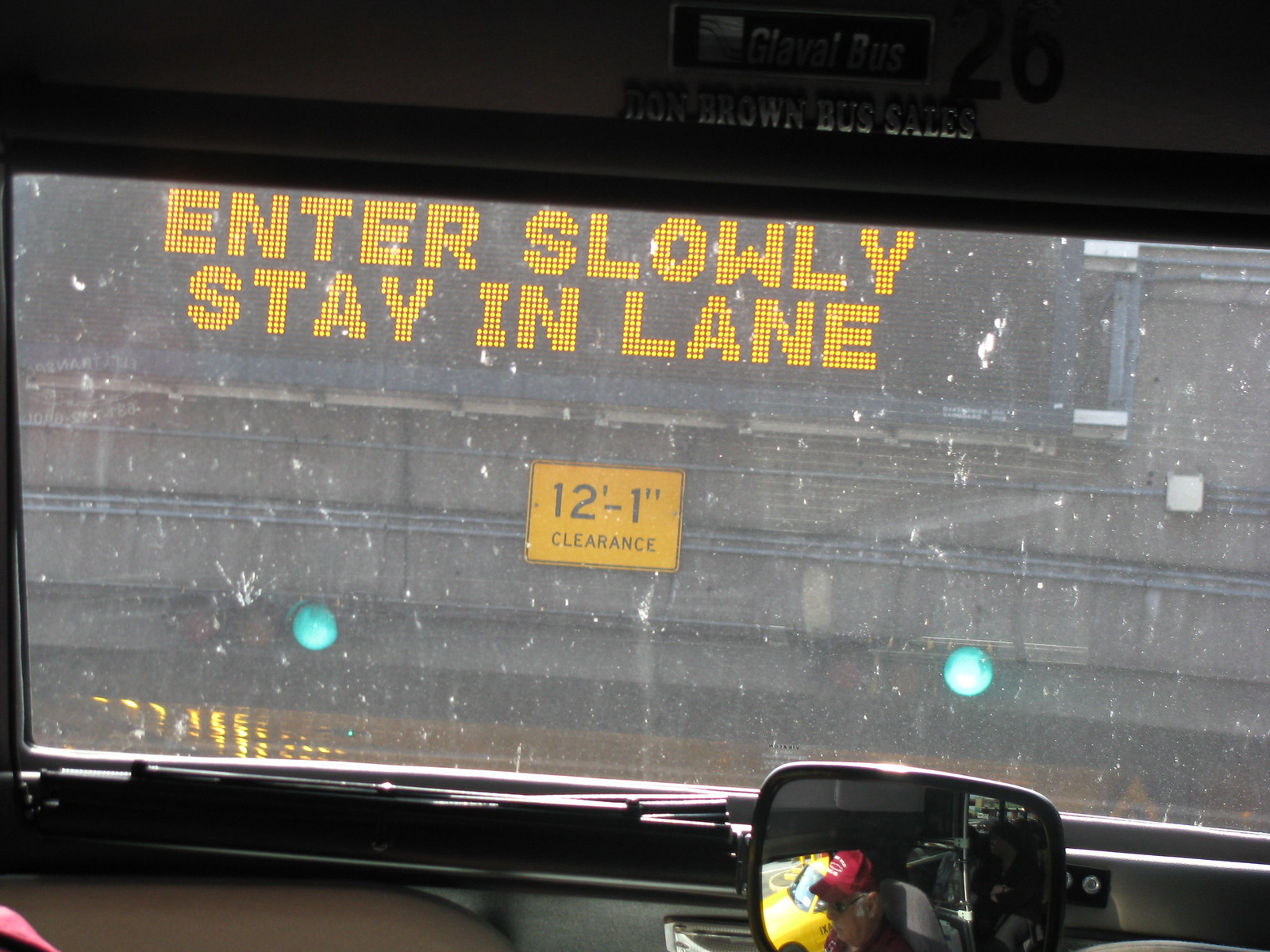A view from inside a bus, looking out through the front windshield on a snowy day. Snowflakes gently cascade, creating a frosted effect on the glass. Around the edges of the windshield, the frame is visible, with a sign at the top reading "Don Brown Bus Sales" in chrome letters. Just above this, a sticker prominently displays the brand "Glavel Bus." To the right of the sticker, the number "26" is visible. In the lower right corner of the image, a rearview mirror reflects the silhouette of the bus driver, adding a human element to this wintry scene.